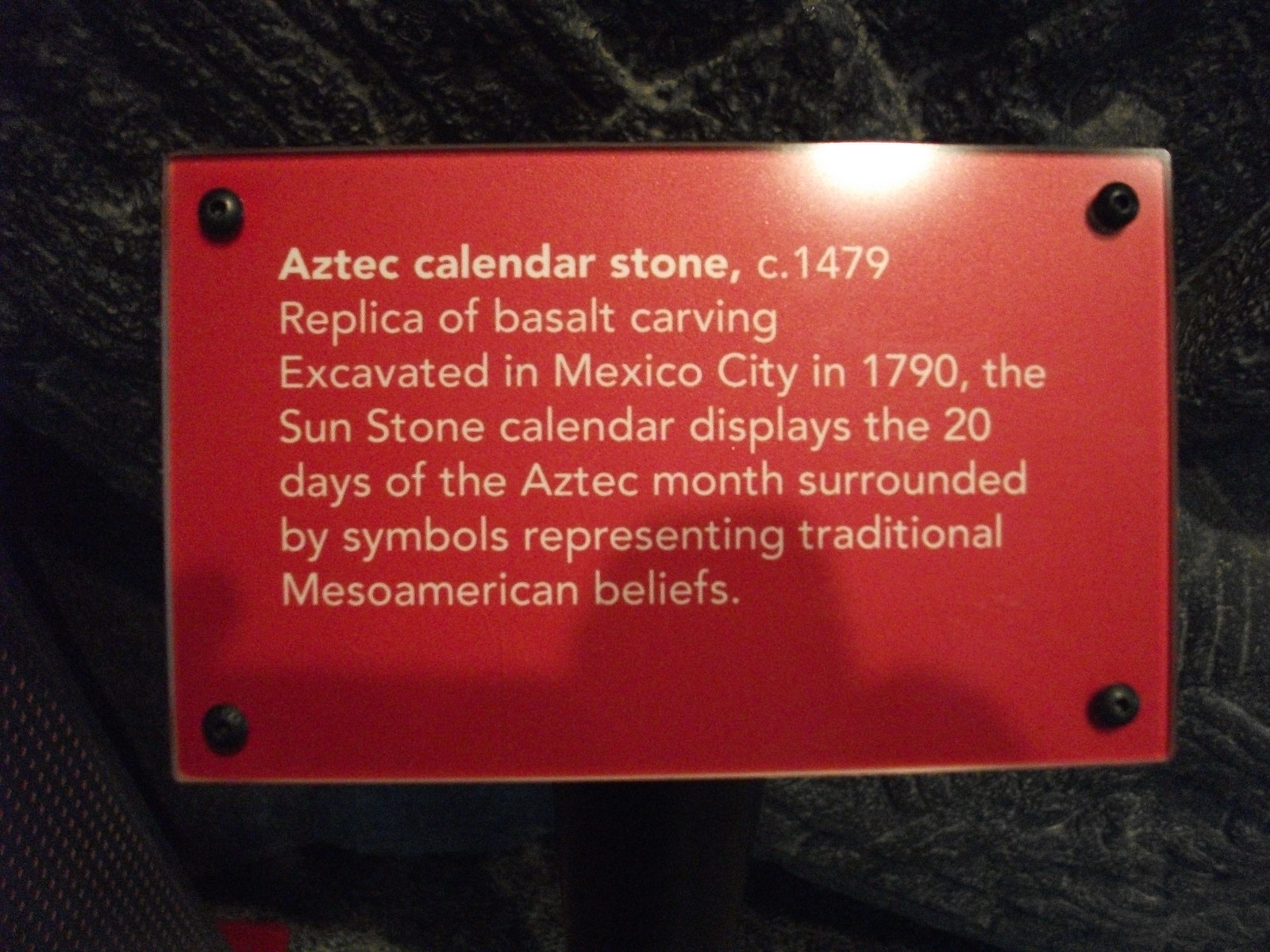This close-up color photograph features a red informational plaque, firmly affixed with four black screws at each corner. The plaque's white text reads: "Aztec Calendar Stone, circa 1479. Replica of basalt carving excavated in Mexico City in 1790." It provides further detail that "The sunstone calendar displays the 20 days of the Aztec month, surrounded by symbols representing traditional Mesoamerican beliefs." The plaque is set against a backdrop of black marble, likely part of a larger display, though the exact nature of this setting—whether indoors or outdoors—remains unclear due to the limited visible context. In the bottom left corner of the image, a netted black material is faintly discernible, adding a subtle layer of texture to the scene. The overall impression is of an artifact display, emphasizing the historical and cultural significance of the Aztec calendar stone while highlighting the meticulous presentation details.